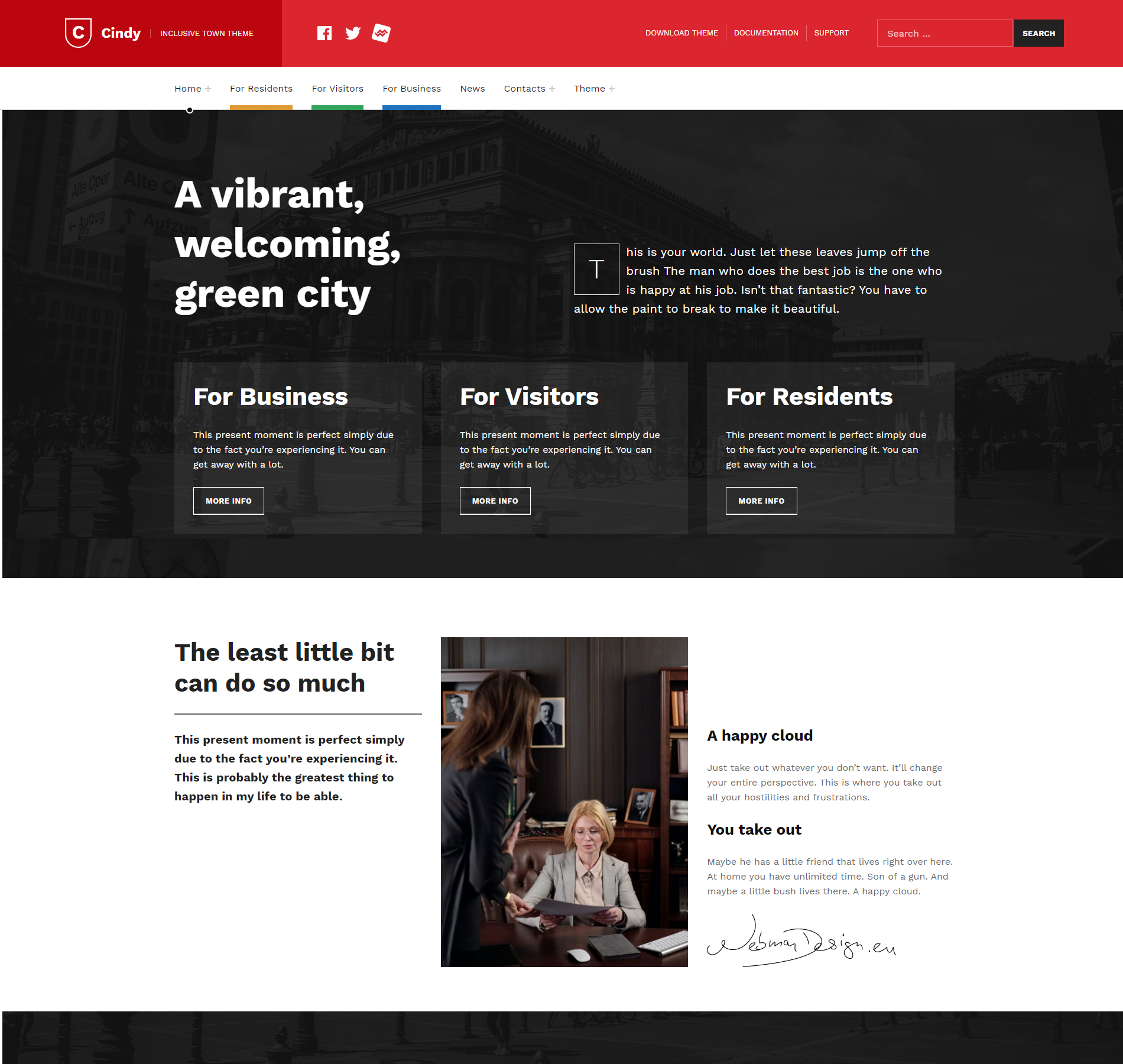This screenshot captures a vibrant, well-organized webpage designed to represent a bustling, welcoming city. At the top of the page, a red bar displays the website's header, featuring a capital "C" on a shield symbol alongside the name "Cindy" in white text. This bar also includes icons for Facebook, Twitter, and an unfamiliar logo, along with options such as "Download Theme," "Doc," an unreadable word, "Support," and a search bar.

Below this header, a white navigation bar with black text offers links to "Home," "For Residents," "For Visitors," "For Business," "News," "Contacts," and "Theme." Dominating the center of the webpage is a bold black rectangle with white text proclaiming "A Vibrant Welcoming Green City." This section includes an inviting paragraph that extols the pleasures of a harmonious work life, emphasizing the joy and creativity involved in painting, likening it to the beauty of the city itself: "This is your world. Just let these leaves jump off the brush. The man who does the best job is the one who is happy at his job. Isn't that fantastic? You have to allow the paint to break to make it beautiful."

Following this inspirational message, the page is divided into three sections catering to different audiences, labeled "For Business," "For Visitors," and "For Residents." Beneath these categories, additional text communicates the sentiment that even the smallest contributions can have a significant impact: "The least little bit can do so much." 

The overall layout and design suggest a community-focused site dedicated to enhancing the experience of its users, whether they are residents, visitors, or business professionals.